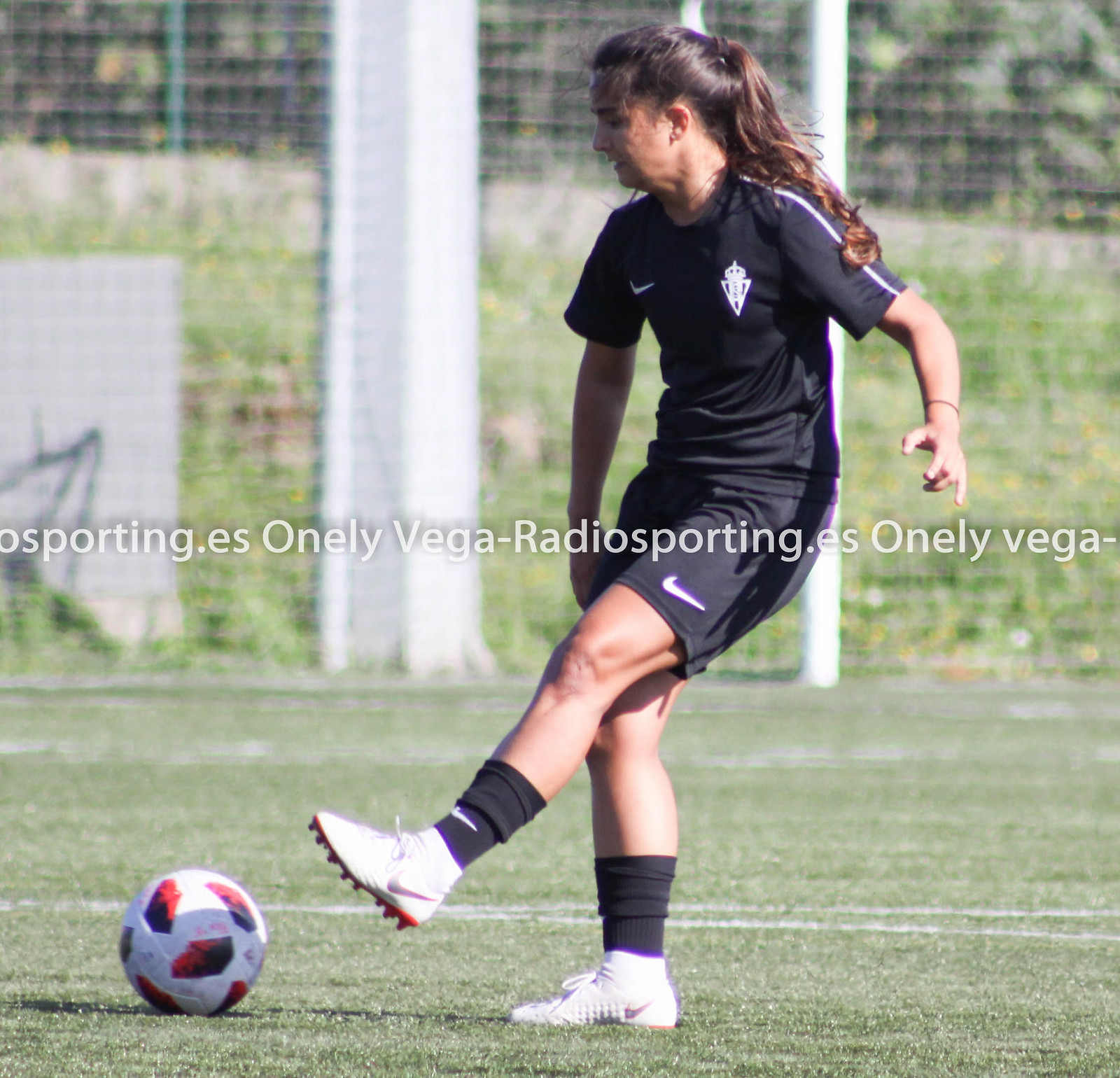In this detailed image, we see a soccer player, likely a woman with long brown hair tied in a ponytail, centered on a soccer field. She's captured in the midst of kicking or having already kicked a white soccer ball adorned with red and black or blue patterns, which is positioned to the right side of the frame. The athlete is donned in a sleek black Nike uniform, including a black shirt, shorts with a Nike stripe, black socks, and white soccer shoes that appear to be Nike-branded as well. The field is marked with white lines, and a large fence can be seen in the background, serving to contain the soccer balls within the playing area. Centrally located within the photo is a gray watermark reading "sporting.es, oneleevega-radiosporting.es."